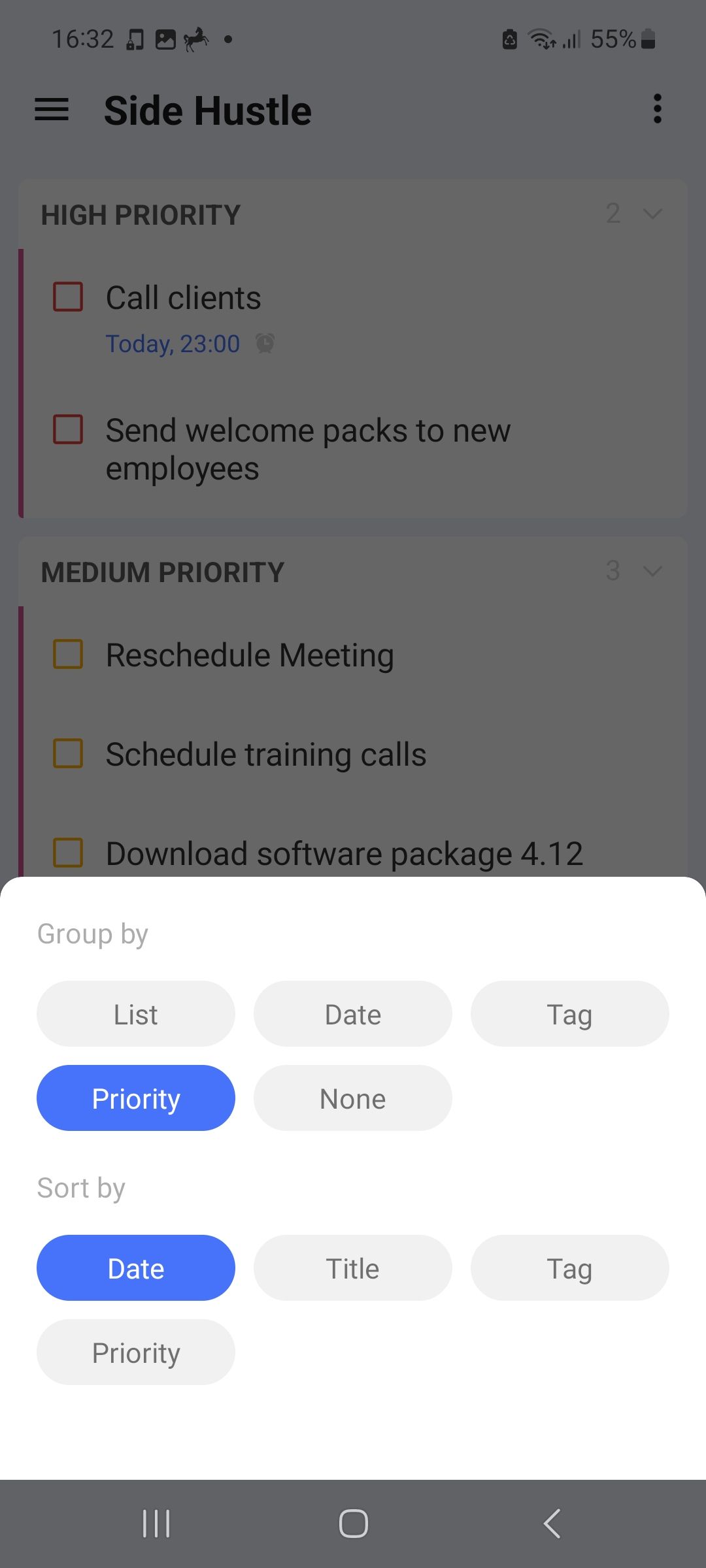This detailed caption depicts a screenshot of a phone displaying a digital to-do list. The current time, shown in the top left corner, is 16:32. The phone's status bar reveals full service signal strength, full WiFi connectivity, and the battery level at 55%.

The title of the checklist, labeled "Side Hustle," is categorized under "High Priority" with two tasks, each marked by a red square checkbox. The first task is to "Call clients today at 2300 hours," and the second task is to "Send welcome packs to new employees."

A secondary section titled "Medium Priority" contains tasks denoted by yellow checkboxes. These tasks include "Reschedule meeting," "Schedule training calls," and "Download software package 4.12."

Below the task lists, the sorting options are detailed, allowing the user to group items by list, date, tag, priority, or none. Additionally, tasks can be sorted by date, title, tag, and priority, ensuring efficient task management.